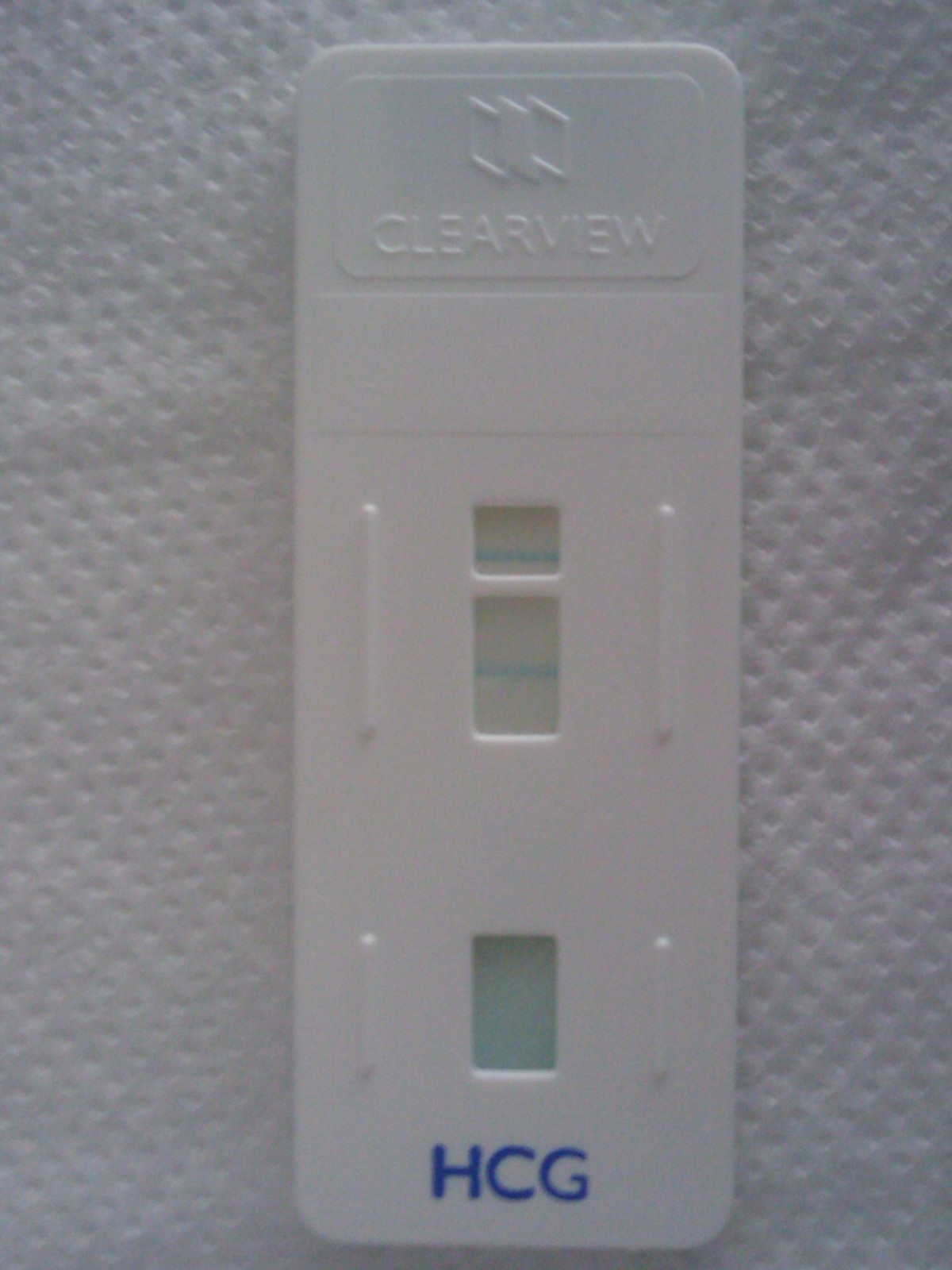The image features a backdrop that appears to be a paper towel, identifiable by the numerous small circular indentations across the white surface, suggesting a thicker material typical of paper towels. Prominently displayed at the top of the image is the brand name "Clear View." The main object in the image is a long rectangular device, approximately 7 inches in length and 3 inches in width. 

Directly below the brand name is a small square with a horizontal light blue line across its center. Following this, there is a longer rectangle situated in the middle, also featuring a horizontal blue line. About 2 inches further down, there is another rectangular section shaded in a muted blue color, devoid of any lines. At the bottom of the device, the bold blue uppercase letters "H-C-G" are clearly visible. 

Based on these features, the object appears to be a Clear View brand pregnancy test. The faint lines and the structured, segmental layout further support this identification. Additionally, white vertical lines are noted on both sides of the squares and rectangles, adding to the item's detailed description.